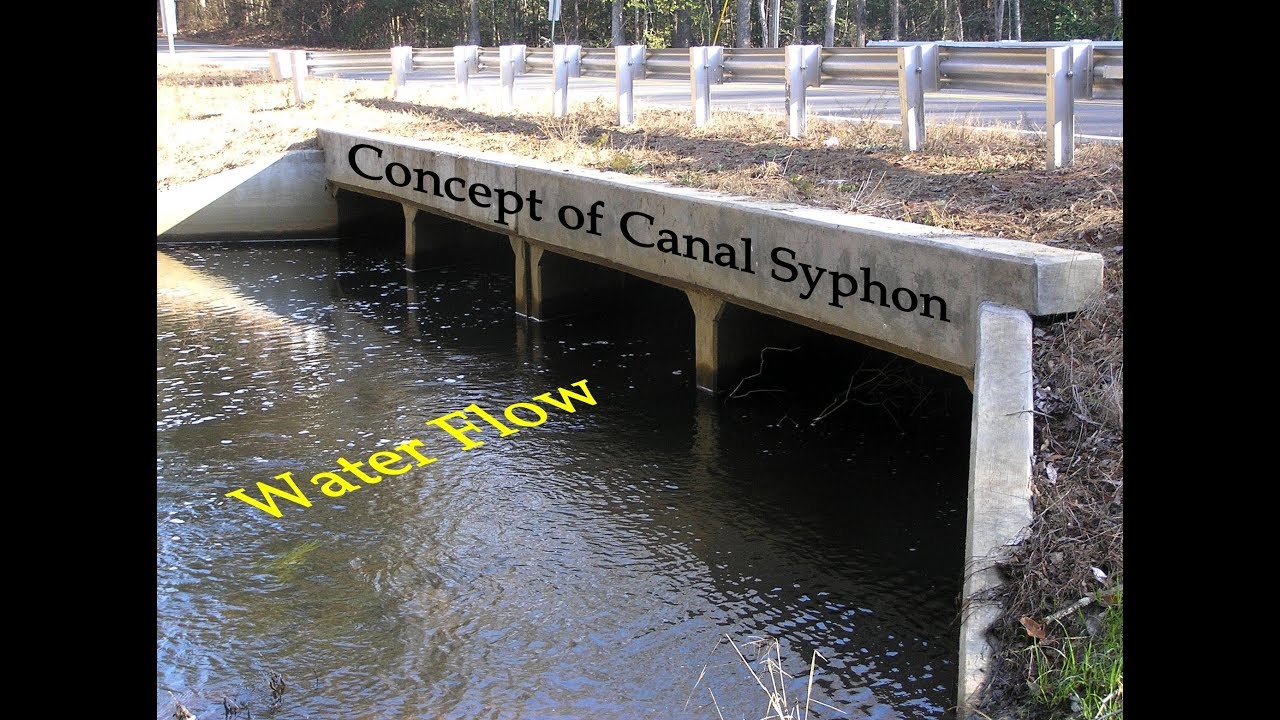This is a detailed, color photograph in landscape mode depicting the concept of a Canal Siphon. The focal point is a concrete and steel bridge, underneath a railway, spanning a brown-colored canal. Text overlays are present, with "Concept of Canal Siphon" in black written on the concrete bridge and "Water Overflow" in yellow marking the water's flow direction. The bridge comprises concrete slabs supporting a larger one, creating a shadowy underpass where the canal flows. Above the bridge, you see a roadway lined with silver metal guardrails, separating the road from the bordering dirt and grass. To the right, there is a patch of grass and dirt next to the concrete structure. The background features a forested area with trees and various plants, adding a natural green backdrop to the scene.